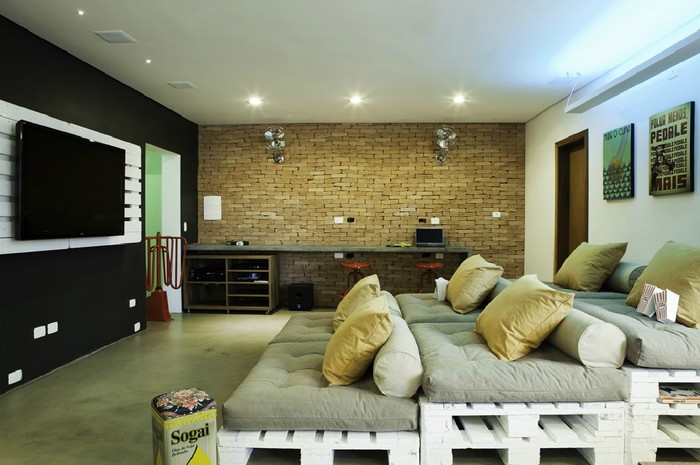This image shows a detailed view of a cozy, DIY media room. The focus is on tiered, custom-built seating made from white-painted stacked pallets. The seating consists of three levels: three pallets on the back row, two in the middle, and one in the front, all topped with gray upholstered cushions. Each level features tan bolsters and bright yellow throw pillows. 

In front of the seating, a large television screen is mounted on a black wall. Below the TV and on either side of the seating, two bowls of popcorn are visible, enhancing the movie-theater feel. To the left of the center bench is a yellow product labeled "Sogueia." 

The room has a polished concrete floor and is bordered by different textured walls: a white wall on the right, a black wall on the left, and a tan-colored brick wall at the back. This back wall also features a brown door with two art pieces hanging above it. Additionally, there's a long desk extending across part of the back wall, adding a functional touch. The ceiling, equipped with three lights, illuminates the space warmly, making it an inviting environment.